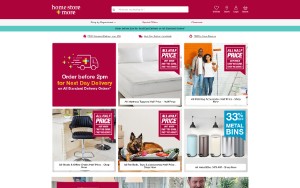This image is a cropped and out-of-focus screenshot of a website's storefront. At the top of the image, there's a prominent red banner featuring a small white search bar centered within it. On the right side of this red bar, you'll find three icons: a heart, a login icon, and a shopping cart. 

Directly beneath the red banner, three category listings are displayed in gray text, followed by a blue bar containing black text, which is too small to read clearly. The main body of the website has a white background and showcases a grid of six fully visible thumbnails.

The top-left thumbnail displays a red box with the text "Order before 2 p.m. for next day delivery." Adjacent to it, there's an image of a bed; this thumbnail also has a red box in the top-right corner with the word "Price" prominently displayed among smaller white text. The thumbnails are organized in two rows of three each. At the bottom edge of the image, the top portions of three additional thumbnails are partially visible but mostly cropped out.